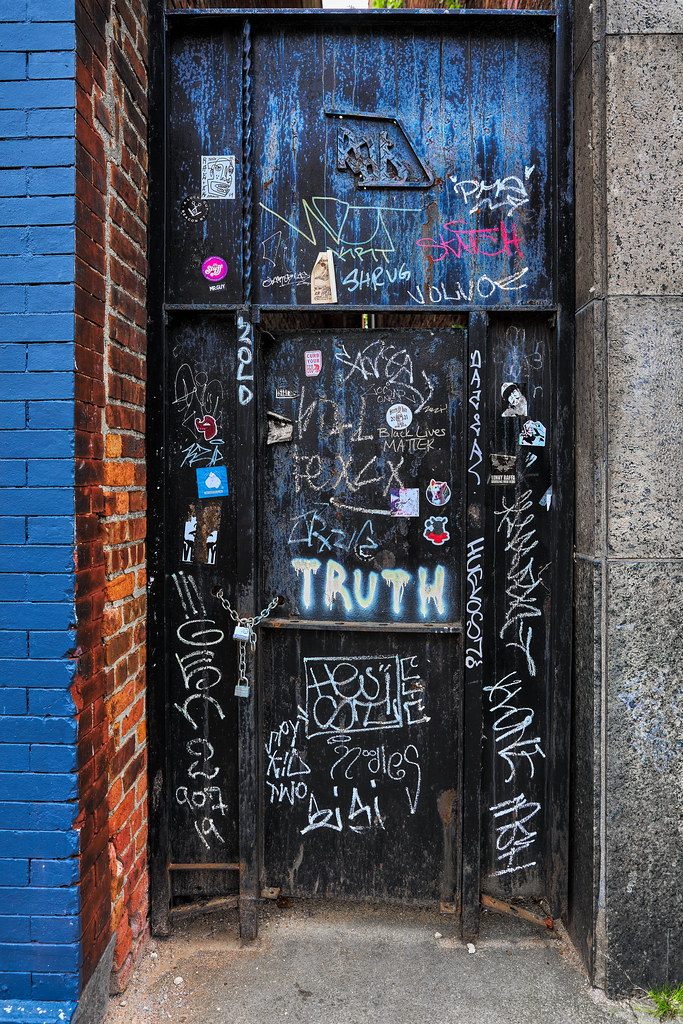This vertical photograph captures an intriguing scene of a doorway that appears to belong to an abandoned building. The door itself is a dark blue or very dark gray, constructed with vertical wooden planks and heavily decorated with an array of graffiti in various mediums, including chalk and paint. Starting from about one-fifth down from the top, the door features random chalk graffiti in white, yellow, and pink, but the text and images are indistinct and unreadable. A wooden divider or support is situated roughly one-third down the door, beneath which the graffiti significantly increases in density.

The most prominent and discernible piece of graffiti, in bold white paint, spells out the word "TRUTH" in all capital letters at the midpoint of the door. Surrounding this are chaotic scribbles and markings, creating a heavily vandalized appearance. Some indications of stickers are also present amidst the graffiti.

The left side of the image is framed by a red brick wall that corners into a perpendicular wall painted blue, adding an element of contrast to the scene. On the right side, the door is framed by a light gray stone wall. The bottom edge of the image shows a gritty and light cement sidewalk with hints of grass peeking through the edges, as well as what could be a chain and padlock, suggesting an attempt to secure the door, possibly to keep vagrants out. The overall aesthetic of the door and its surroundings indicate an area that has been neglected over time, with vivid graffiti and signs of wear contributing to its dilapidated charm.